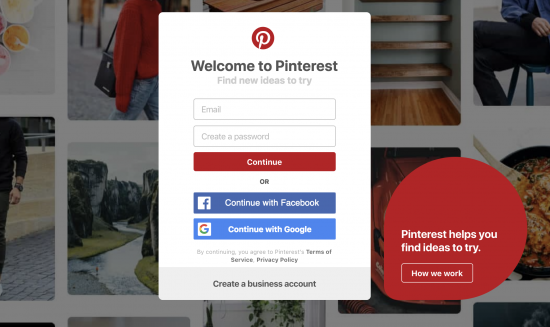**Detailed Caption:**

The image is a screenshot of the Pinterest login screen. Central to the screen is a prominent white login window. At the very top of this window is the Pinterest logo: a red circle with a stylized, white script "P" inside. Directly underneath the logo, bold text reads "Welcome to Pinterest." Below this greeting is a line of gray text that encourages users to "Find new ideas to try."

Further down, users are invited to log in by entering their credentials. Two vertically aligned fields, one labeled "Email" and the other "Create a Password," are outlined with thin gray lines. Situated beneath these input fields is a large red button labeled "Continue." 

Users are also presented with alternative login options. The options are prefaced by the word "Or" and feature two blue buttons: "Continue with Facebook" and "Continue with Google," each accompanied by their respective icons to the left.

Towards the bottom of the window, a brief disclaimer states, "By continuing, you agree to Pinterest’s Terms of Service and Privacy Policy."

Finally, at the base of the white window in a gray bar, there is an option to "Create a Business Account." Adjacent to this in the bottom right corner is a red, circular button reiterating that "Pinterest helps you find new ideas to try."